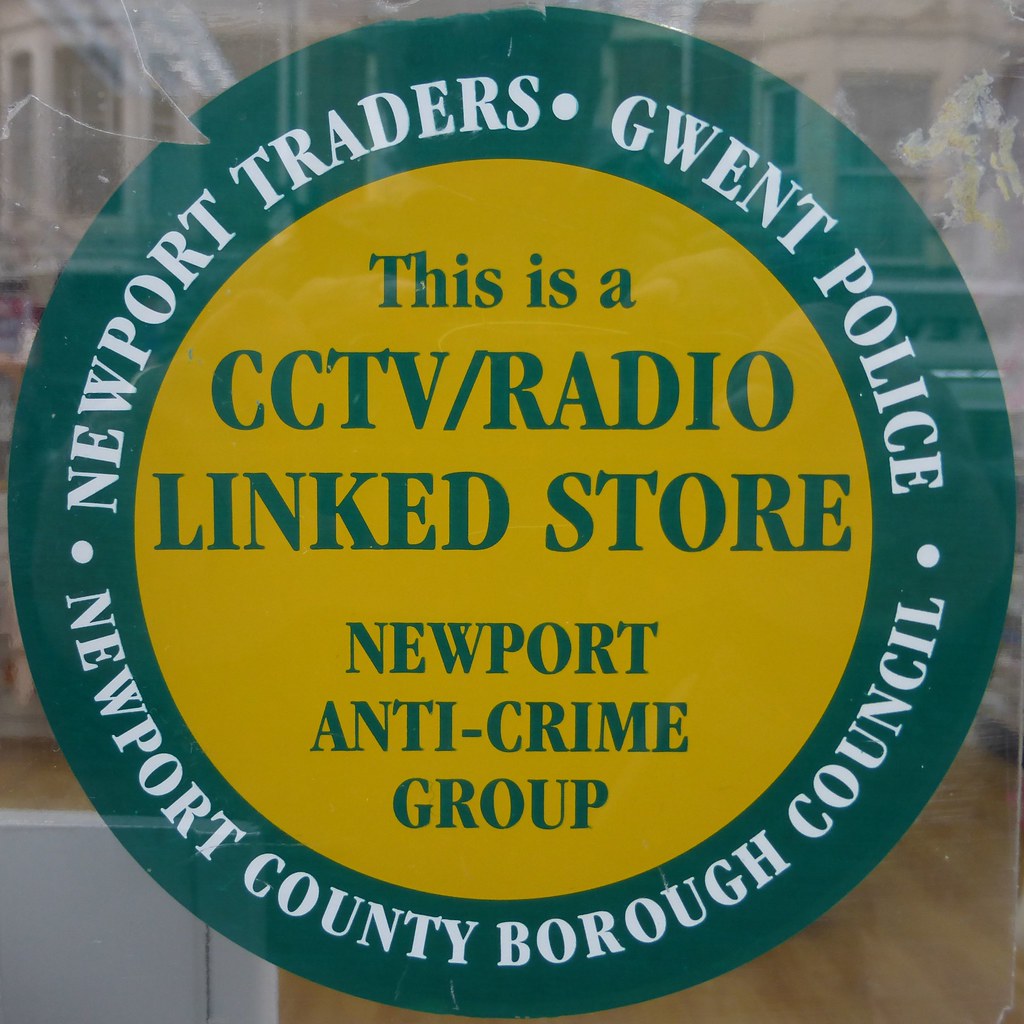This photograph captures a slightly cracked window pane, with the crack visible in the upper left corner. Adhered to the window is a round sticker, prominently detailed with an aqua blue border. In white text around the border, the sticker reads "Newport Traders, Gwent Police" at the top and "Newport County Borough Council" at the bottom. At the center of the sticker is an olive-colored circle with blue text that states, "This is a CCTV radio linked store. Newport Anti-Crime Group." The window is somewhat reflective, revealing a blurred view of a wooden floor inside the store and faint reflections of houses in the background. The image is highly detailed, focusing on the circular sign and the minor crack on the glass.